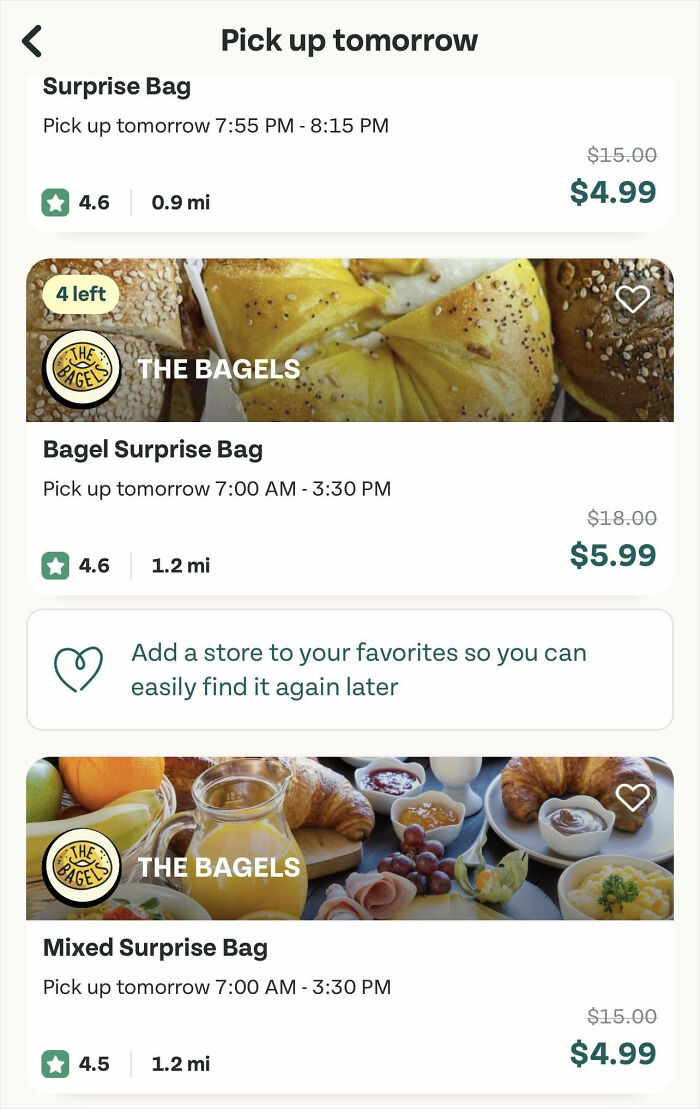This screenshot captures the interface of an application or website designed to offer surprise bag options for pickup. The background is predominantly white, creating a clean and minimalistic look. 

At the top center of the screen, the heading "Pick Up Tomorrow" is prominently displayed. To the left of this heading, there is a left-pointing arrow, likely for navigating back to the previous screen. 

Just below the main heading, in bold black text on a white background, it reads "Surprise Bag." It further specifies, "Pick Up Tomorrow, 7:55 PM to 8:15 PM." Beneath this section, there is a green logo featuring a white star in the middle, accompanied by a rating of "4.6" stars and a distance indicator showing "0.9 miles." Adjacent to this in red text is a price reduction from "$15" to "$4.99" highlighted in green.

Following this information, an image of bagels appears with a description indicating there are "4 left." It details a "Bagel Surprise Bag" available for pickup from 7:00 AM to 3:30 PM. The rating for this bag is "4.6" stars, and the distance is specified as "1.2 miles." The price listed is "$5.99."

Below this, a prompt encourages users to "Add A Store to your favorites so you can easily find it again later," enhancing usability and user convenience.

Further down the screen, there is another business logo or item listing labeled "the bagels." This section features a picture of croissants accompanied by a plate of fruits, vegetables, and a large mug of orange juice. The caption for this part states "Mixed Surprise Bag," available for pickup from 7:00 AM to 3:30 PM. The rating is "4.5" stars, situated "1.2 miles" away, with a listed price of "$4.99."

Overall, the screenshot showcases various surprise bag options with corresponding ratings, distances, and prices, providing a clear and user-friendly interface for potential customers.